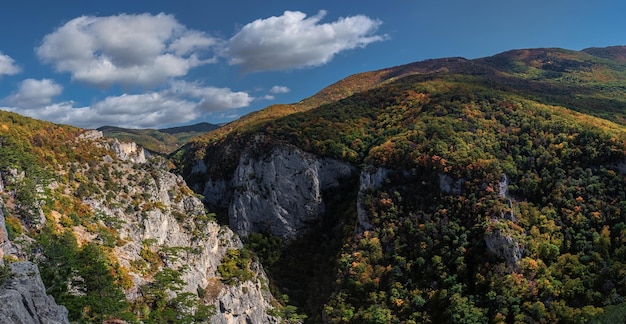The image captures a breathtaking mountain landscape under a vivid blue sky adorned with puffy white clouds. In the background, majestic mountains rise into the horizon, creating a sense of vastness and awe. The foreground features rolling hills to the right, densely populated with trees displaying a vibrant spectrum of foliage in varying shades of dark green, bright green, yellow, and brown, indicative of the changing seasons.

Dominating the middle ground is a prominent rocky cliff, its rugged gray surface enhancing the scene's dramatic natural beauty. The terrain suggests the presence of a hidden valley, shrouded by a dense canopy of trees, hinting at a depth and mystery that invites closer exploration.

To the left, another rocky mountain ascends, sporadically cloaked with trees in hues of green, yellow, and brown. The summit is marked by a mix of green and brown, contrasting sharply with the rockier lower slopes. The overall impression is one of serene, untouched wilderness, devoid of any human habitation, with the valley floor remaining out of sight, adding to the scene's enchanting and mysterious allure.